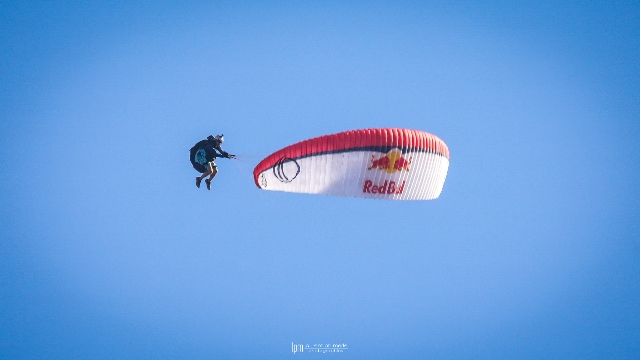In this striking photograph, we see a person skydiving, distinctly mid-air against a backdrop of a vivid blue, cloudless sky. They are wearing a helmet, shorts, sneakers, and a dark backpack-like gear. Notably, their parachute, which is not deployed above them but rather in front and parallel to their body, features prominent Red Bull branding. The parachute displays a vivid red top section with the signature Red Bull logo - a yellow circle with two red bulls charging towards each other. Beneath the logo, "Red Bull" is written in bold red letters. A black line divides the upper red part from the lower white section, which includes blue outlines and circles. This unusual configuration suggests the person is performing a stunt, as they appear to be positioned as if sitting upright, with the parachute acting almost like a windshield. The sky's subtle gradient - lighter at the center, darker at the triangular corners - frames the dynamic action of the scene. White, barely discernible text or symbols can also be seen at the bottom, likely a time stamp or a signature.